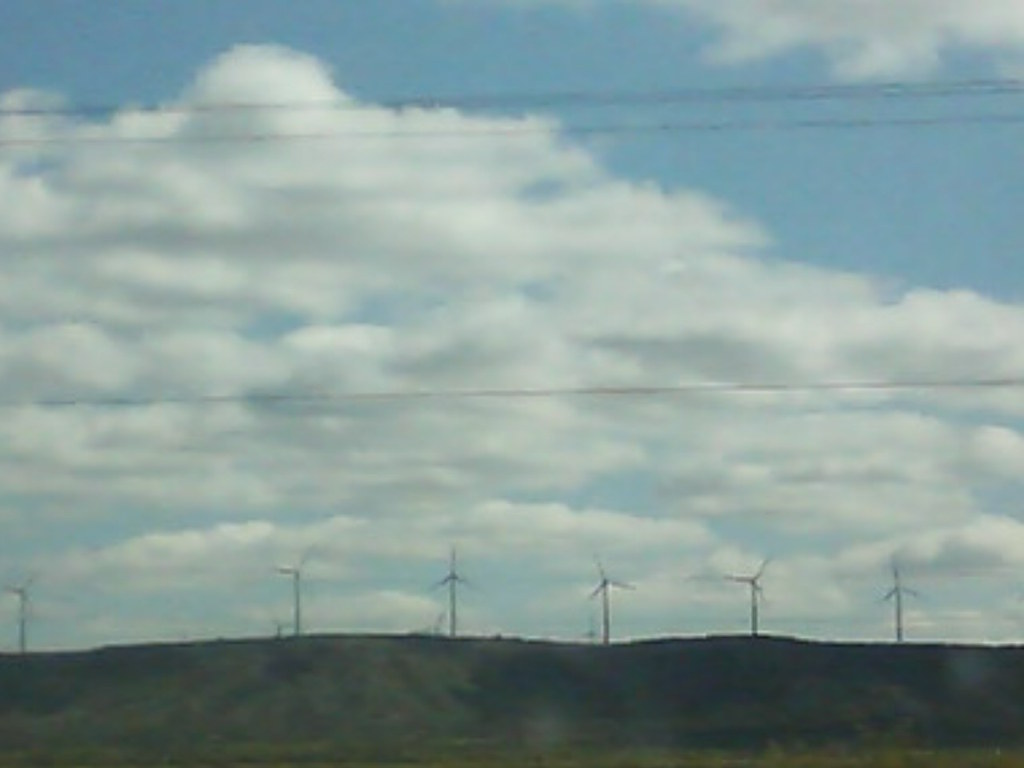This image is a very blurry color photograph, likely taken from inside a moving vehicle such as a train or car. Dominating the majority of the image is a sky with flat white and slate gray clouds. There is a noticeable cyan tint to the photograph, which may suggest it is an old film photograph converted to digital form. Stretching across the sky are three thin wires, possibly telephone or electrical wires, positioned along the center and top portions of the image. In the upper background, the sky is filled with out-of-focus, fluffy clouds. The foreground, however, remains an indistinct dark green, almost black shadowed area that reveals no details. Along the horizon line at the base of the image, there are six windmills, white in color, with vertical support posts and three-bladed rotors, evenly spaced to capture wind energy. Despite the challenge in discerning the exact size of these windmills due to the lack of scale reference, they are a distinct feature on the gently rolling hill at the bottom of the picture.